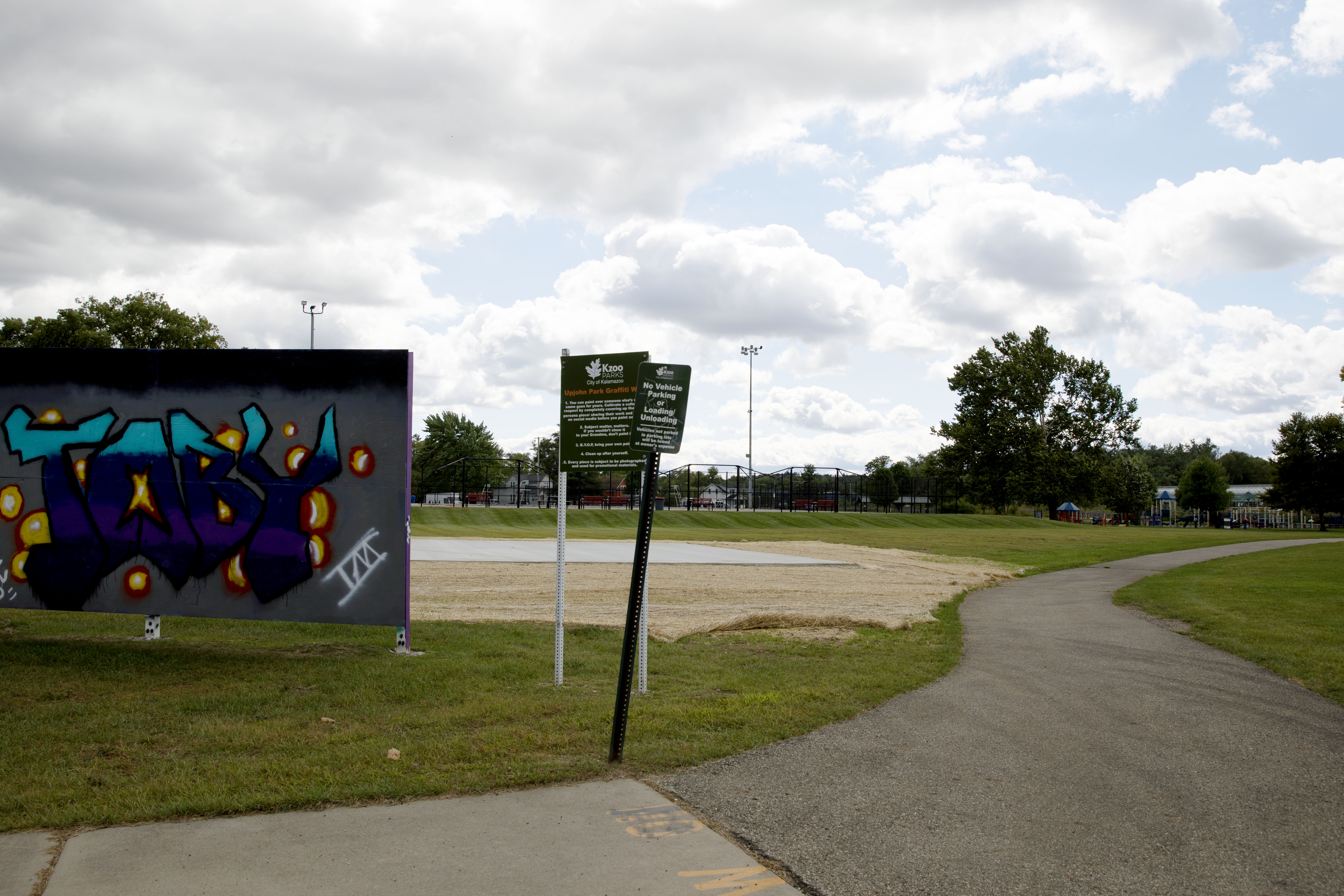This image depicts the entrance of a public park, highlighting a paved sidewalk that winds through the foreground and curves off to the right. Flanking the sidewalk is a neatly mown grassy area adorned with two signs bearing white letters on a green background, one of which reads "No Vehicle Parking." To the left stands a concrete wall, embellished with colorful graffiti that spells out "Toby" in shades of blue with yellow bubbles behind it. A fence, large trees, and playground equipment are visible in the distance, along with a baseball diamond situated towards the center of the image. The cloudy sky, filled with thick clouds, stretches across the background, adding a muted, bluish-gray hue to the overall scene.